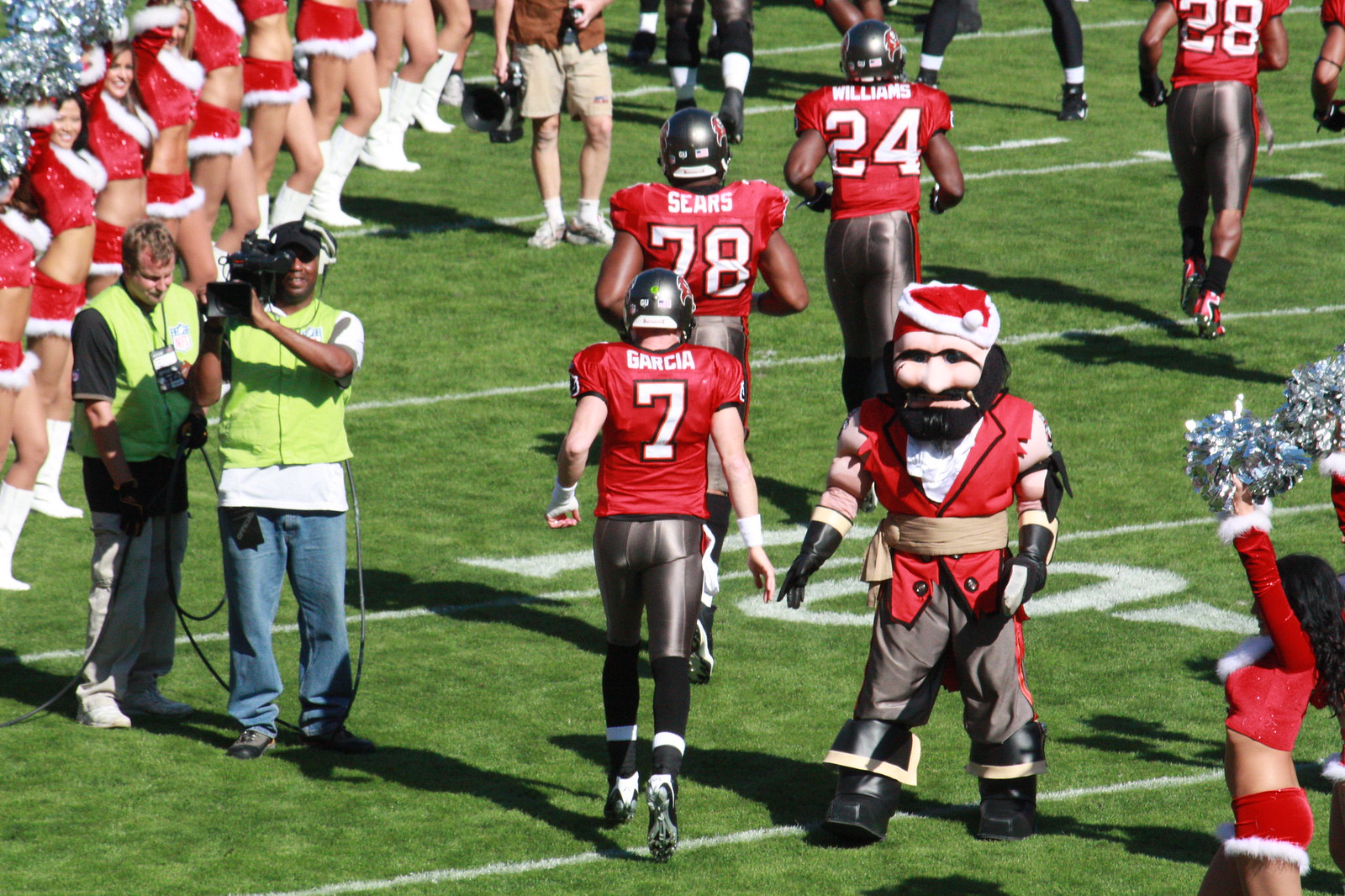The image captures a vibrant football event set outdoors in the middle of the day on a large, grassy field with marked lines. In the upper left corner of the photo, a squad of cheerleaders enthusiastically supports the team. Adjacent to them are two cameramen in bright lime-green vests; one holds cables and the other a camera. The center of the image is dominated by football players, identifiable by their red jerseys and tight gray pants, running towards the back. Prominently nearby player number 7 is the team's mascot, dressed in a nautical-themed costume featuring gray slacks, a semi-formal red shirt, white collar ruffles, small black-gloved hands, and a Santa hat. The photo features a vivid array of colors, including green, white, lime green, red, gray, brown, and black. The scene is full of energy and color, emphasizing the excitement of the event.